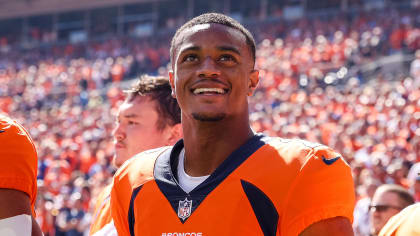The photograph captures a joyful moment of an African American football player, who appears to play for the Denver Broncos, given his orange jersey with black details and blue highlights. The jersey features a Nike swoosh on the shoulder and a small NFL logo in the middle of the v-neck. The player is smiling up at the scoreboard, suggesting he sees something that makes him happy. Surrounding him are other teammates also clad in orange jerseys, their faces and profiles visible. Behind them, the image blurs to reveal a packed stadium filled with fans, predominantly wearing orange, indicating the likelihood of a home game. Above the stands, windows of indoor seating sections are visible. The atmosphere suggests an important game, possibly a championship, adding to the significance of his elation.